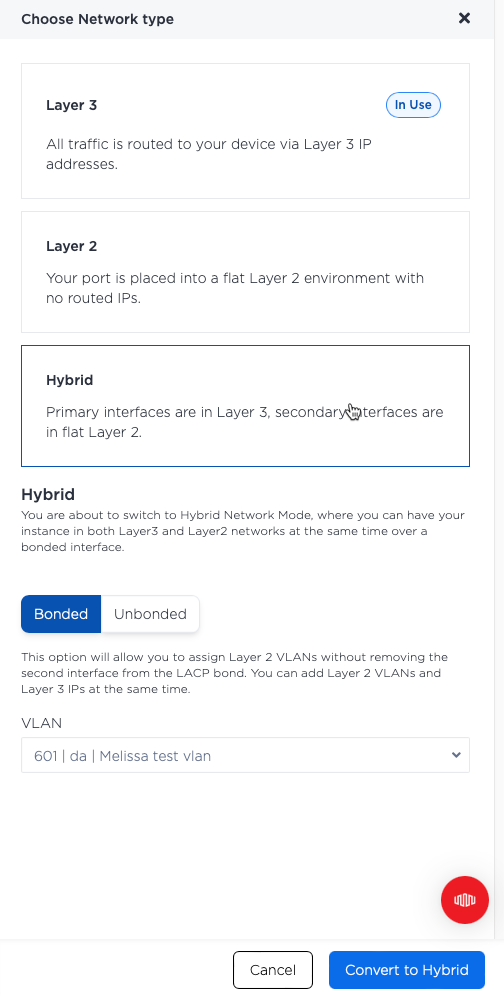The image features a network selection page with a comprehensive interface for choosing and configuring network modes. 

At the very top, a light gray header strip reads "Choose Network Type." Directly below this, there is a section labeled "Layer 3," which explains, "All traffic is routed to your device via Layer 3 IP addresses." To the right of this description, a blue button labeled "In Use" indicates that Layer 3 is currently active.

Following this section is the "Layer 2" option, stating, "Your port is placed into a flat Layer 2 environment with no routed IPs."

Beneath these options, there's a bordered rectangle containing the word "Hybrid." It details, "Primary interfaces are in Layer 3. Layer interfaces are in flat Layer 2." A cursor, represented by a hand icon, points precisely at the 'I' in "interfaces."

Further down, the page elaborates on the Hybrid mode, with a message that reads, "You are about to switch to Hybrid network mode where you can have your instance in both Layer 3 and Layer 2 networks at the same time over a bonded interface."

Below the descriptive text are two rectangular buttons: one with a blue background labeled "Bonded," and another with a white background labeled "Unbonded."

A subsequent explanatory note says, "This option will allow you to assign Layer 2 VLANs without removing the second interface from the LACP bond. You can add Layer 2 VLANs and Layer 3 IPs at the same time." It also includes the word "VLAN" followed by a text box containing numbers and words for user input.

At the very bottom of the page, there are two additional action buttons: a gray rectangle labeled "Cancel" and a blue rectangle labeled "Convert to Hybrid."